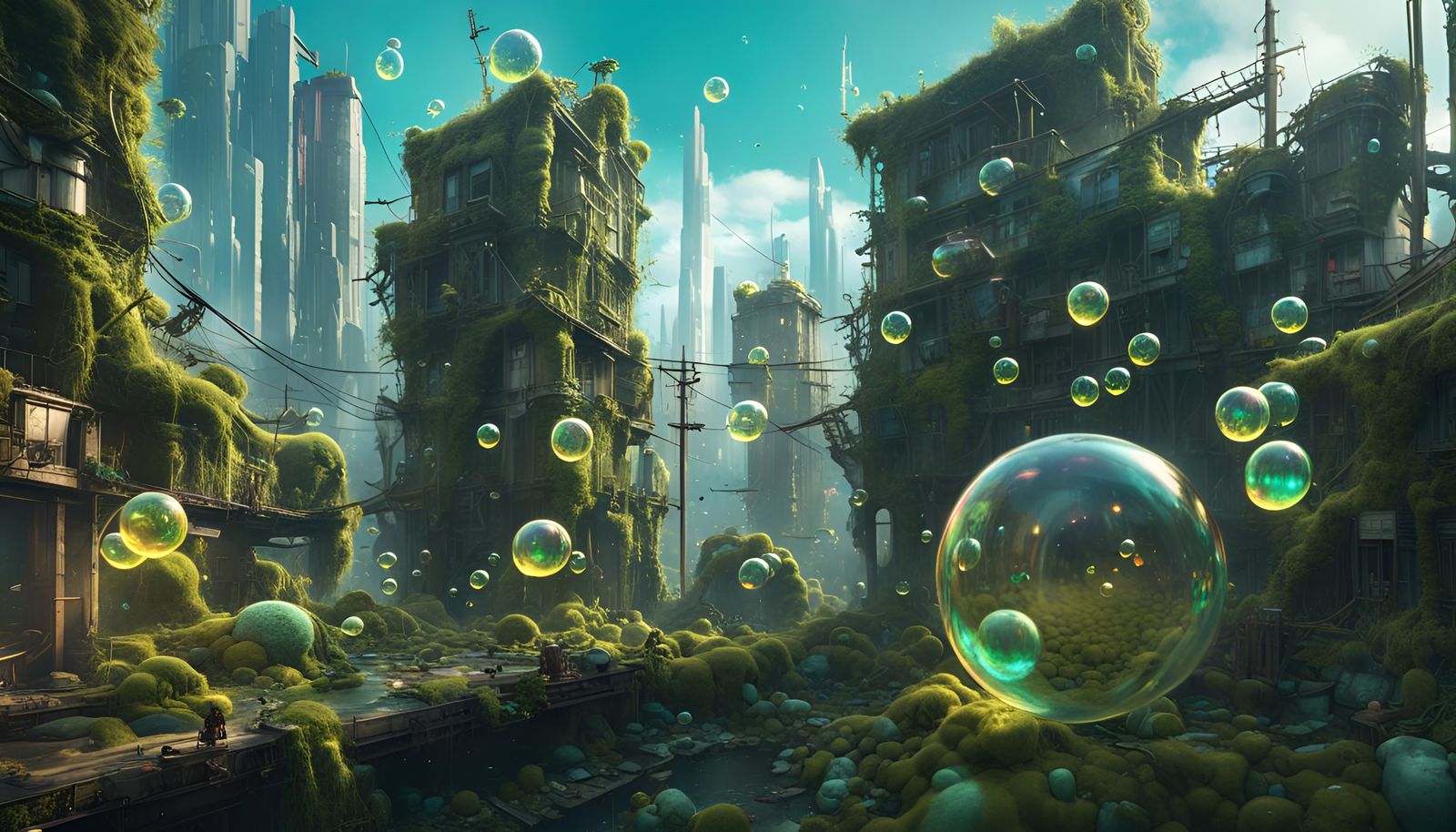The image depicts a digital AI-generated drawing of an apocalyptic city that seems partially submerged underwater, indicated by the numerous bubbles floating in the foreground, varying in size from large to small. The cityscape is derelict and abandoned, its structures crumbling and overgrown with moss and ferns. Three prominent buildings in the front are particularly detailed, showcasing the extent of decay and natural overgrowth. The ground is scattered with moss-covered pebbles, further emphasizing the city's abandonment. In stark contrast, the background reveals a futuristic city with sleek, towering skyscrapers that reach towards the light blue sky, punctuated with white clouds, creating a juxtaposition between the old, moss-covered ruins and the advanced urban skyline.